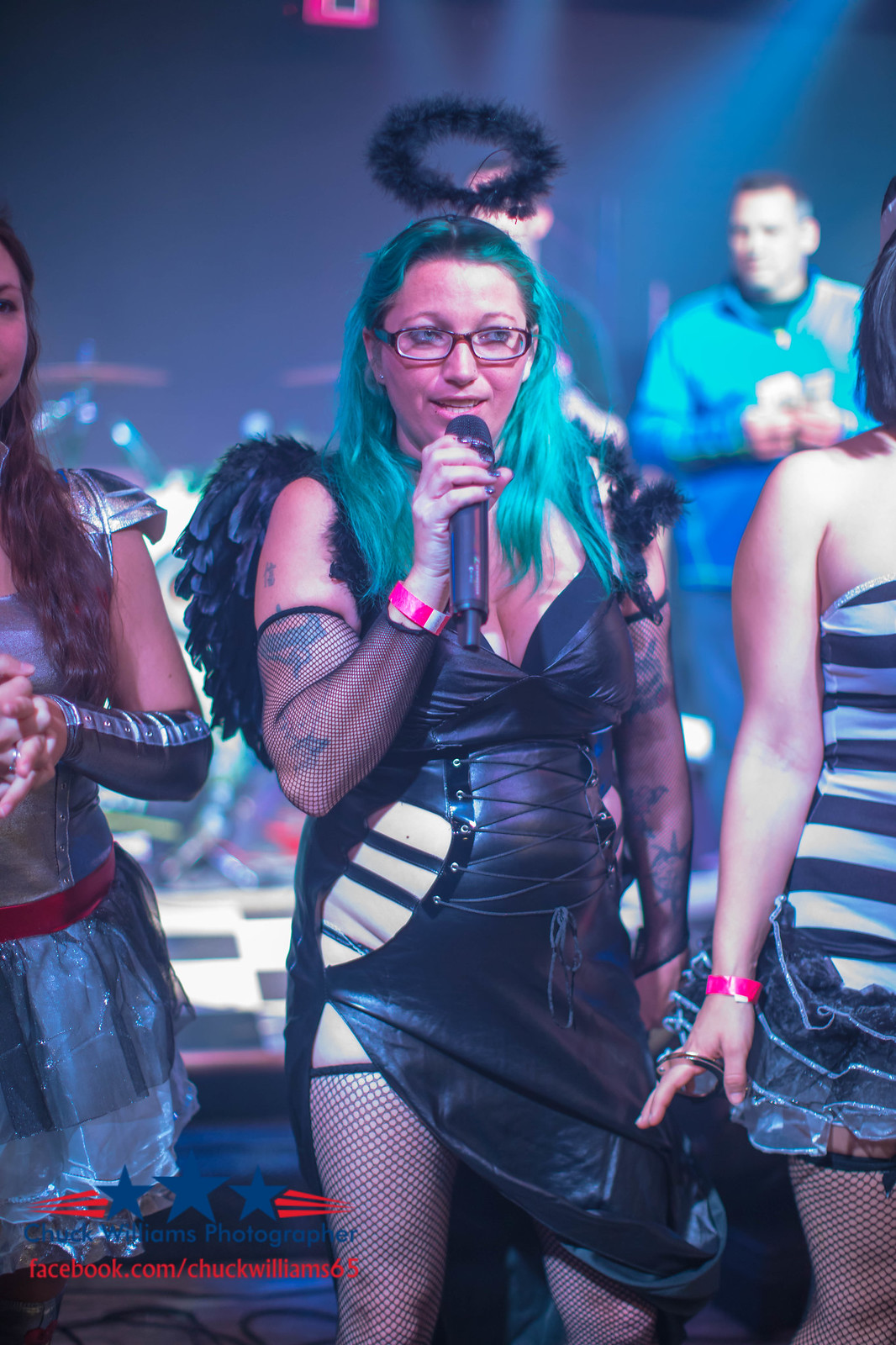The image depicts a lively stage performance featuring a central figure, a slightly heavyset woman, who commands attention. She is adorned in a striking black leather garment that slants downward from her left thigh to her right, revealing her bare right leg clad in fishnet stockings. Her right arm, tattooed beneath a net sleeve, is raised as she holds a microphone to her mouth, her gaze directed slightly to the right. Her vivid turquoise hair cascades over her shoulders, and she sports brown-rimmed glasses. Behind her, a set of feathered wings is visible, contributing to her ethereal stage presence, complemented by a dark greenish wreath above her head.

To her right stands a woman with shoulder-length dark hair, bare shoulders, and a horizontally black and white striped top. A magenta bracelet adorns her right wrist, and her fishnet stockings are revealed through her slightly visible thigh and knee. To the left of the central woman is another performer with long dark brown hair draped over her chest, wearing a light blue frilly dress with a silver strip on her forearm and what appears to be a gray epaulette on her left shoulder.

The background features a dark blue setting with indistinct elements, possibly drums, suggesting a musical performance. A blurred man, clad in a blue jumpsuit and appearing to clap his hands, is visible behind the central figure, adding to the dynamic atmosphere of the scene. The overall composition and attire of the women suggest a thematic and coordinated performance, with each detail contributing to the theatrical and captivating image.